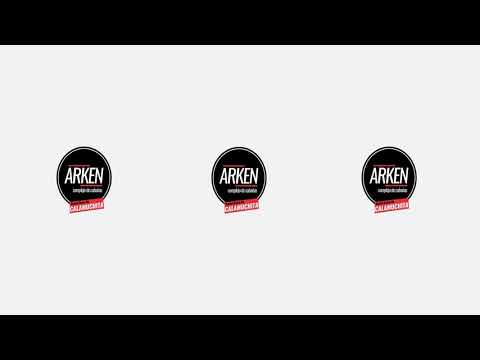The image is a business advertisement set on a wide vertical, rectangular white background, framed by black horizontal stripes at the top and bottom. Positioned evenly across the center, there are three identical black circular logos, each outlined with a slim white ring creating a narrow white gap. Inside each circle, the bold and slightly narrow sans-serif text "ARKEN" is displayed in white. Beneath this text in each logo, there's a small red rectangle angled slightly, also containing unreadable white text. Additionally, there is small, illegible grey text below the main "ARKEN" text within each logo.